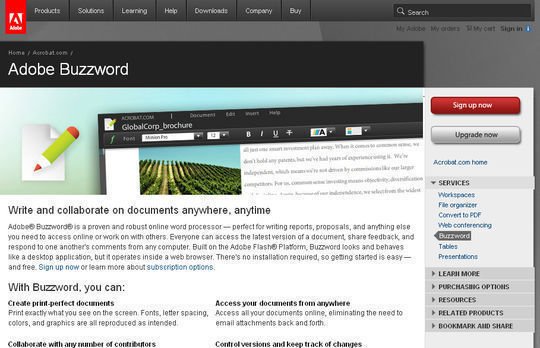This horizontal screenshot features an Adobe webpage with a user interface designed for promoting Adobe Buzzword. The Adobe logo, showcasing its signature white and red colors, is positioned at the top left corner. Adjacent to the logo on the right is a dark grey navigation bar containing options labeled as follows: Podcast or Products, Solutions, Learning, Help, Downloads, Company, and Buy. The top right corner houses a search bar for user convenience.

Below this header section, the webpage background transitions to grey. A horizontal black strip with the text "Adobe Buzzword" in white spans across the top. Along the right-hand side column, there are prominent buttons urging users to "Sign Up Now" in red or "Upgrade Now" in silver. Additionally, some blue-colored links are available for further navigation. Within the open Services tab, Buzzword is highlighted in grey, drawing attention to this specific feature.

The main content area showcases a graphic featuring a green, red, and white pencil overlaid on a piece of paper. This visual is accompanied by a snapshot of another webpage at the top left corner, depicting a scenic photograph of fields under a blue sky. Directly beneath this image, a large section of text reads: "Write and collaborate on documents anywhere, anytime." Following this statement, the text elaborates with the phrase: "With Buzzword you can," and lists four key points:
1. Create print-perfect documents.
2. Collaborate with any number of contributors.
3. Access your documents from anywhere.
4. Control versions and keep track of changes.

This detailed layout effectively communicates the capabilities and benefits of using Adobe Buzzword for document creation and collaboration.